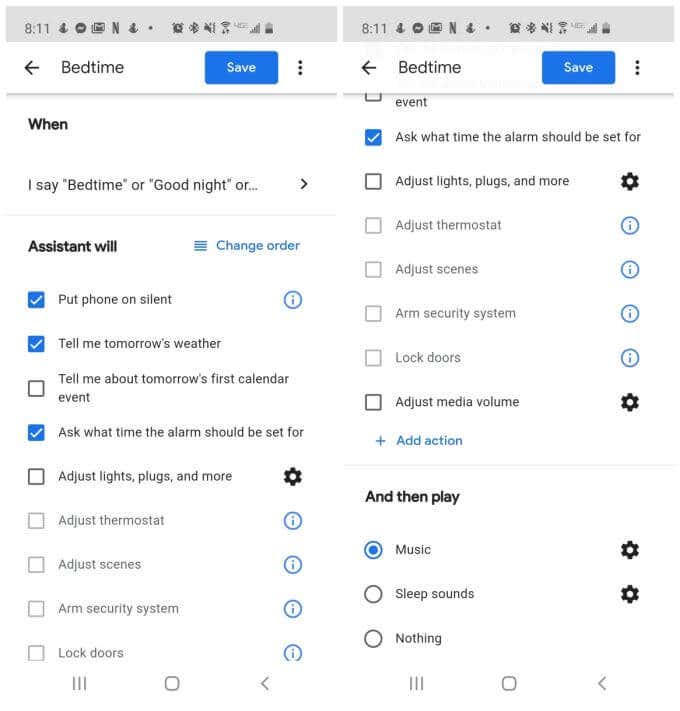The image consists of two screenshots captured from a mobile device, displaying the various options available for configuring a bedtime routine. These options are part of a feature designed to assist users in establishing bedtime settings and automating tasks using their device assistant. 

The first screenshot outlines how users can initiate bedtime mode through voice commands, such as saying "bedtime" or "goodnight." It lists several actions that the assistant can perform when bedtime mode is activated, and the selected options include: 

- Putting the phone on silent.
- Informing the user about tomorrow's weather.
- Asking the user what time the alarm should be set for.

The second screenshot continues listing other potential bedtime actions that have not been selected, which include:

- Providing details about the user’s first calendar event for the next day.
- Adjusting lights, plugs, and other connected devices.
- Modifying the thermostat settings.
- Altering home scenes or automations.
- Arming the security system.
- Locking the doors.

Overall, the screenshots present a comprehensive look at how users can personalize their bedtime routine using their mobile device assistant, offering a range of convenient, automated functions to enhance their nighttime and morning experience.